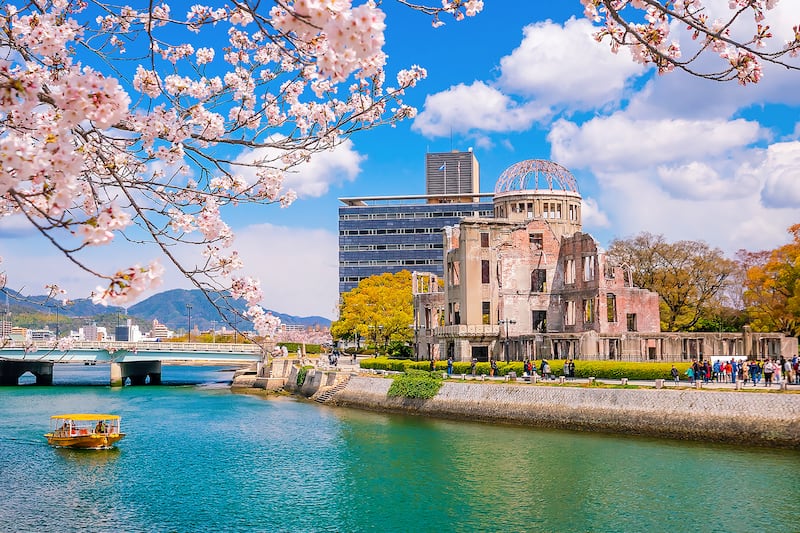The image captures a picturesque landscape featuring a harmonious blend of natural and architectural elements, evocative of an Asian setting, possibly Japan. Dominating the center of the image are two distinct buildings. One in the far distance showcases a dome-shaped roof, while another, blue in color with numerous windows and a rectangular design, stands prominently. Closer to the viewer, an ancient, partially ruined structure with brown and red hues hints at a storied past. 

To the left of the image, lush, vegetation-covered mountains or hills interspersed with a few buildings rise against a backdrop of a vibrant blue sky dotted with scattered white clouds. Cherry blossom trees with delicate light pink petals and intricate branches adorn the upper portion of the image, particularly more prevalent on the left side, adding an elegant and classically Japanese touch.

A tranquil body of water reflecting green and teal hues spans the lower section, featuring a yellow boat with passengers and a bridge to the bottom left of the image. In the lower right corner, several people are visible, going about their daily activities amidst green vegetation.

The overall composition creates a serene yet dynamic atmosphere, merging the beauty of nature with historical and modern architectural splendor.